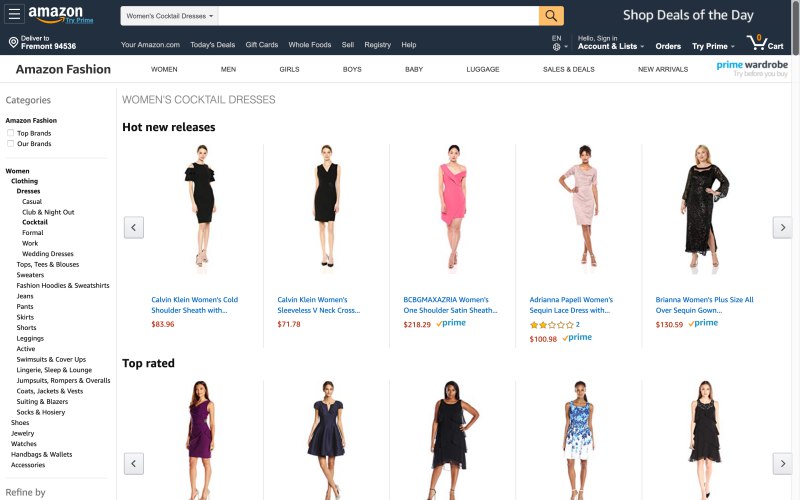### Descriptive Image Caption:

This image captures an Amazon shopping page set to deliver to Fremont, ZIP code 94536. The top-left corner displays the Amazon menu with three horizontal lines and following sections: "Your amazon.com," "Today's Deals," "Gift Cards," "Whole Foods," "Sell," "Registry," and "Help." Positioned above the search bar, the interface highlights options such as "Shop deals of the day," "Hello, sign in," "Accounts & Lists" (with a drop-down menu), "Orders," "Try Prime" (also a drop-down menu), and "Cart (0)."

The product display is focused on women's dresses. At the top, an image of a model showcases a Calvin Klein women's cold shoulder sheath dress priced at $83.96, though the text is partially cut off. Below it, another Calvin Klein dress, a sleeveless V-neck cross style, is listed at $71.78. Both dresses are black.

Further down, a pink BCBG Max Azria women's one-shoulder sheath dress is available for $118.29. Another dress, this time a light pink Adrianna Papell women's sequin lace dress, is priced at $100.98 and rated two stars from two reviewers. This item includes a Prime check mark, indicating eligibility for Prime shipping.

Lastly, a black Brianna women's plus size all-over sequin gown is shown, priced at $130.59 with a Prime check mark. Beneath these listings, images of additional dresses feature models wearing dresses in colors such as purple, blue, black, black-and-white, and black once again. 

This detailed depiction highlights the various options and price points for women's dresses available on Amazon.